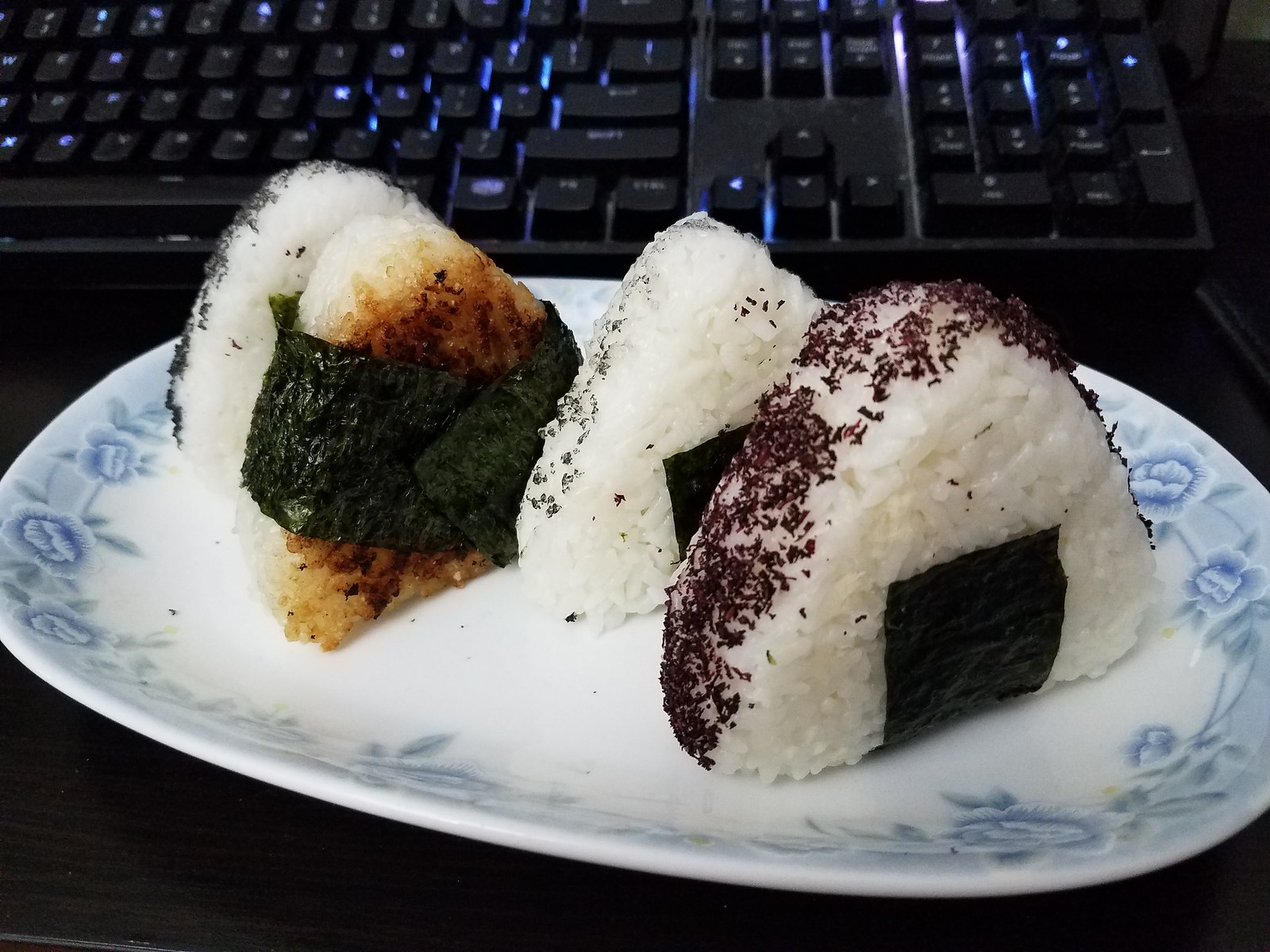This photograph features a meticulously arranged plate of Japanese vegetarian sushi, specifically triangular rice shapes inspired by onigiri. Each of the four pieces differs slightly in appearance, showcasing the uniqueness and artistry of the preparation. The rice triangles are neatly wrapped with nori seaweed that forms a door-like appearance on what resembles a miniature igloo. The forefront piece is adorned with a brown spice or herb crust, while the adjacent white one features a different seasoning encrusting it. A third piece, darker and fully enveloped in seaweed like a shawl, appears to have been cooked longer, giving it a rich brown hue. The final piece behind is similar to the second one, maintaining the visual balance. These sushi pieces are set on a white, oval-shaped bowl with a delicate light blue floral pattern. This charming bowl rests on a sleek black wooden desktop, with a glimpse of a black computer keyboard illuminated by blue backlight subtly visible in the background, hinting at a healthy lunch break amidst work.